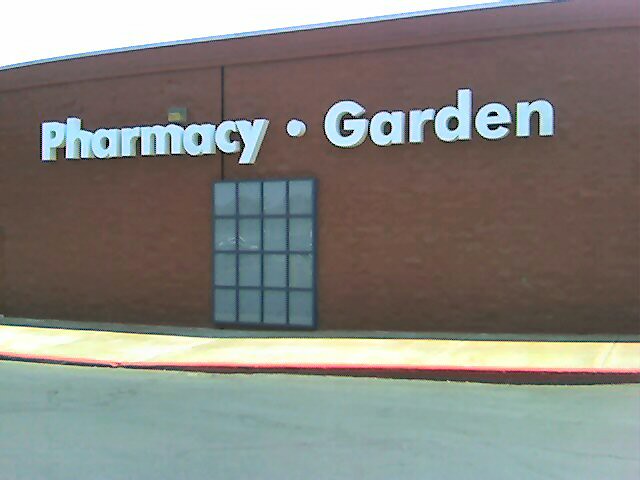This color photograph shows the exterior of a large, chocolate brown building with the words "Pharmacy" and "Garden" prominently displayed in large white font, with a small white dot between them. Below the text, a notable feature is the large, frosted white window, framed in dark blue, which consists of 16 smaller rectangular panes. In front of the building lies a yellowy white sidewalk with a red curb separating it from the gray asphalt of the parking lot. Above the building, a gray line runs along the top, and to the left of the "M" in "Pharmacy," there is an indiscernible black object with a yellow smudge.